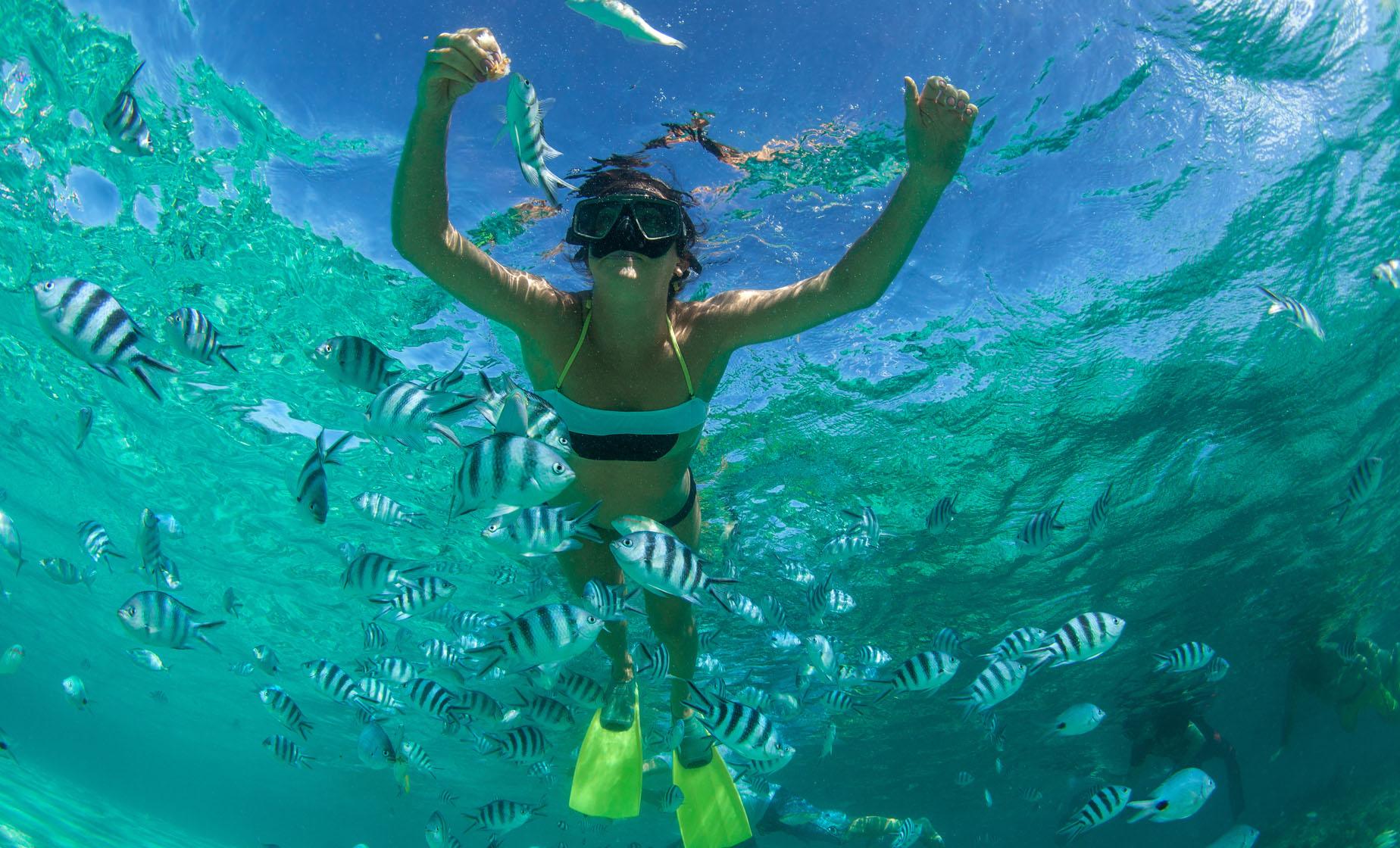In this underwater photograph, a woman is captured swimming in what appears to be the ocean. She is wearing a white and black bikini, bright yellow fins, and a snorkeling mask over her eyes, but not her mouth, suggesting she is holding her breath. Her arms are fully extended in front of her as she floats just below the surface, where sunlight from the morning sky creates bright, dappled patterns on one side and darker shades on the other. Both above and around her, numerous small, black and white striped fish swim in every direction, some even appearing to be interested in something she is holding in her fingers, possibly fish food. The waves can be seen crashing above her, completing this serene yet dynamic underwater scene.